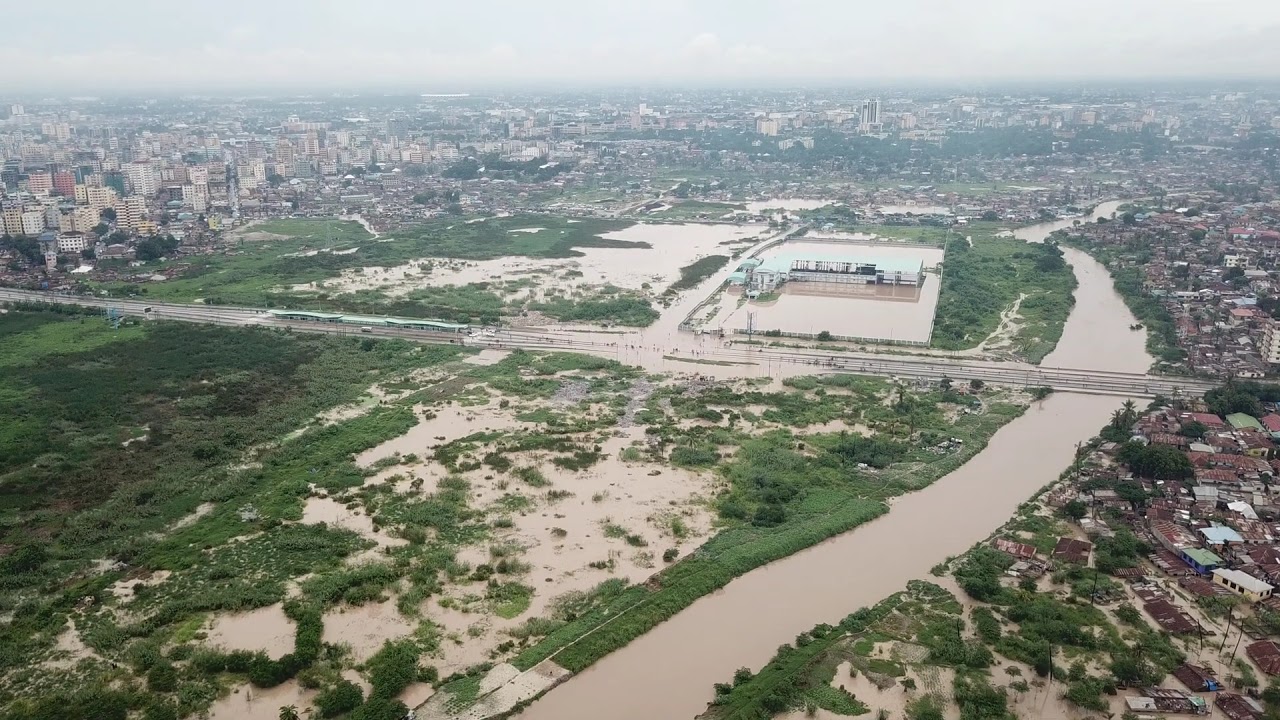This aerial photograph captures a sprawling urban park intersected by a meandering, light brown river, which flows calmly without any ripples. The river originates from the center of the image, curves slightly to the right, veers back towards the center, and then sharply bends right before disappearing off the edge of the frame. On the right side of the river, there's a dense collection of varied buildings, indicative of a residential suburb with houses and smaller structures. On the opposite side, the park features abundant green vegetation interspersed with patches of light brown soil. Notably, in the middle of the park area, there is a prominent white commercial building, possibly a warehouse with a light green roof, surrounded by muddy, dark brown waters, suggesting flooding.

A significant roadway bisects the scene, stretching from the right edge to the left, slightly angled upward. It spans the river via a bridge, appearing inundated with water at several points. The roadway is accompanied by lines of smaller roads crisscrossing the landscape, connecting various buildings scattered across the park and towards the larger city in the background.

The metropolitan backdrop is dense with infrastructure, including tall skyscrapers and shorter commercial and residential buildings, contributing to a stark contrast between the verdant parkland and the urban expanse. The horizon is marked by a hazy sky filled with gray and white clouds, with patches of blue sky faintly visible, reinforcing a subdued and overcast atmosphere in the sprawling cityscape.